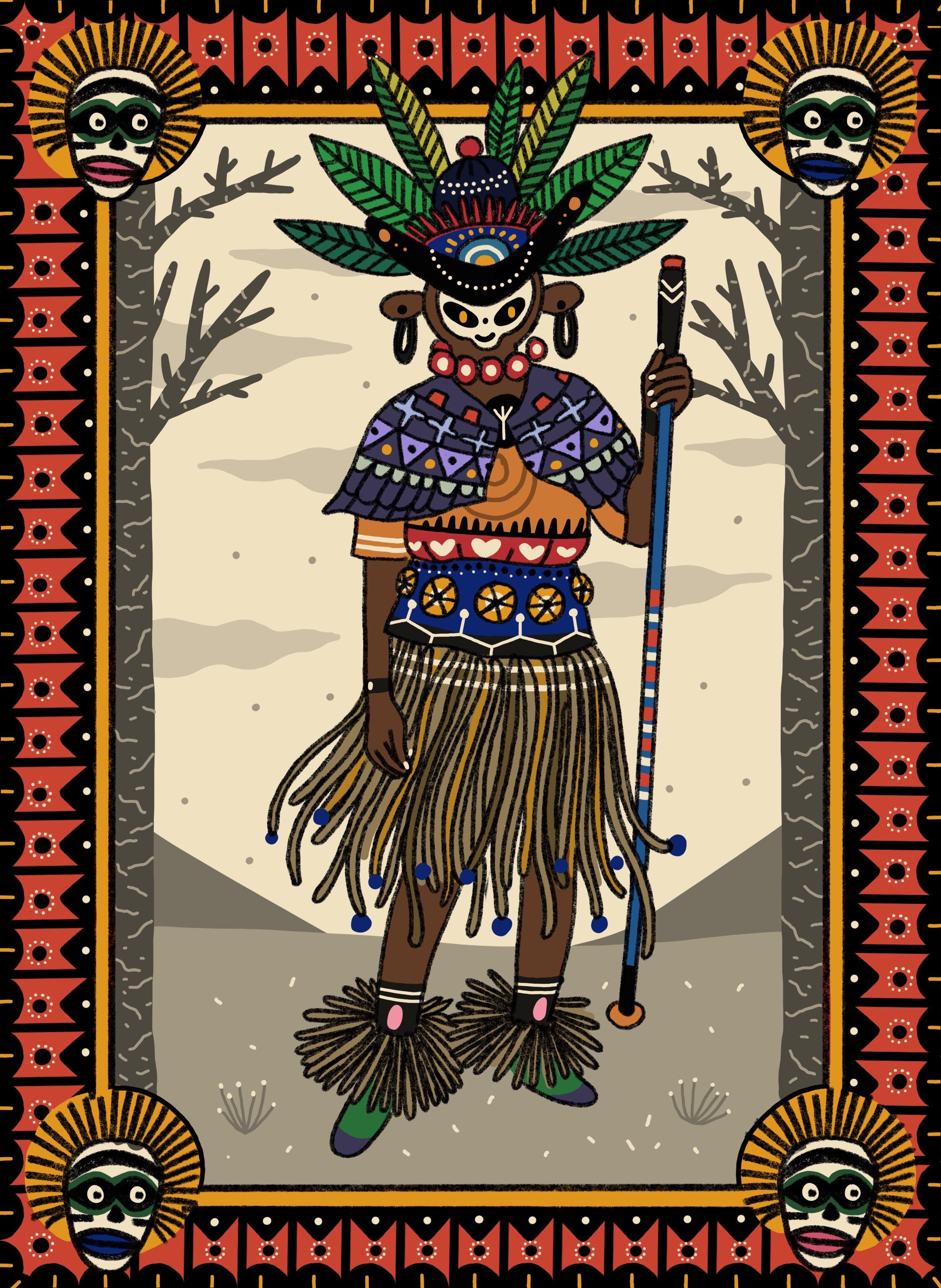The artwork depicts an exotic figure adorned in elaborate, tribal-inspired attire. The central figure wears a white mask with distinctive black eyes featuring yellow dots, and a small nose and mouth. Long ears extend from the head, each adorned with black ring earrings. Above the mask, green leaves with black lines point in various directions. The figure is further accessorized with a striking necklace composed of red beads, with white dots.

The outfit includes a heavy cape draped over the shoulders, setting a dramatic contrast against a predominantly purple background decorated with triangles and yellow dots. Below, a blue waist-high skirt is adorned with yellow circles intersected by black lines. The skirt has long strands of hair hanging below knee level, each tipped with a blue bead. The figure's footwear is green shoes with blue tips, surrounded by circular tufts of hair at the ankles, each with a pink dot.

In the figure's right hand, they hold a blue cane with a black handle and alternating red and white dots along its length. The entire scene is framed by an orange-bordered pattern of square segments with indentations. Each corner of the border features a white face encircled by a yellow ring, marked with green eye circles and differently colored lips—pink in the upper left and lower right, and blue in the upper right and lower left.

The background is a striking contrast with gray trees and a sky filled with various shades of gray clouds, adding to the otherworldly aura of the depicted figure. The overall composition evokes a mixture of tribal and possibly otherworldly aesthetics, reminiscent of motifs associated with African or even voodoo themes.